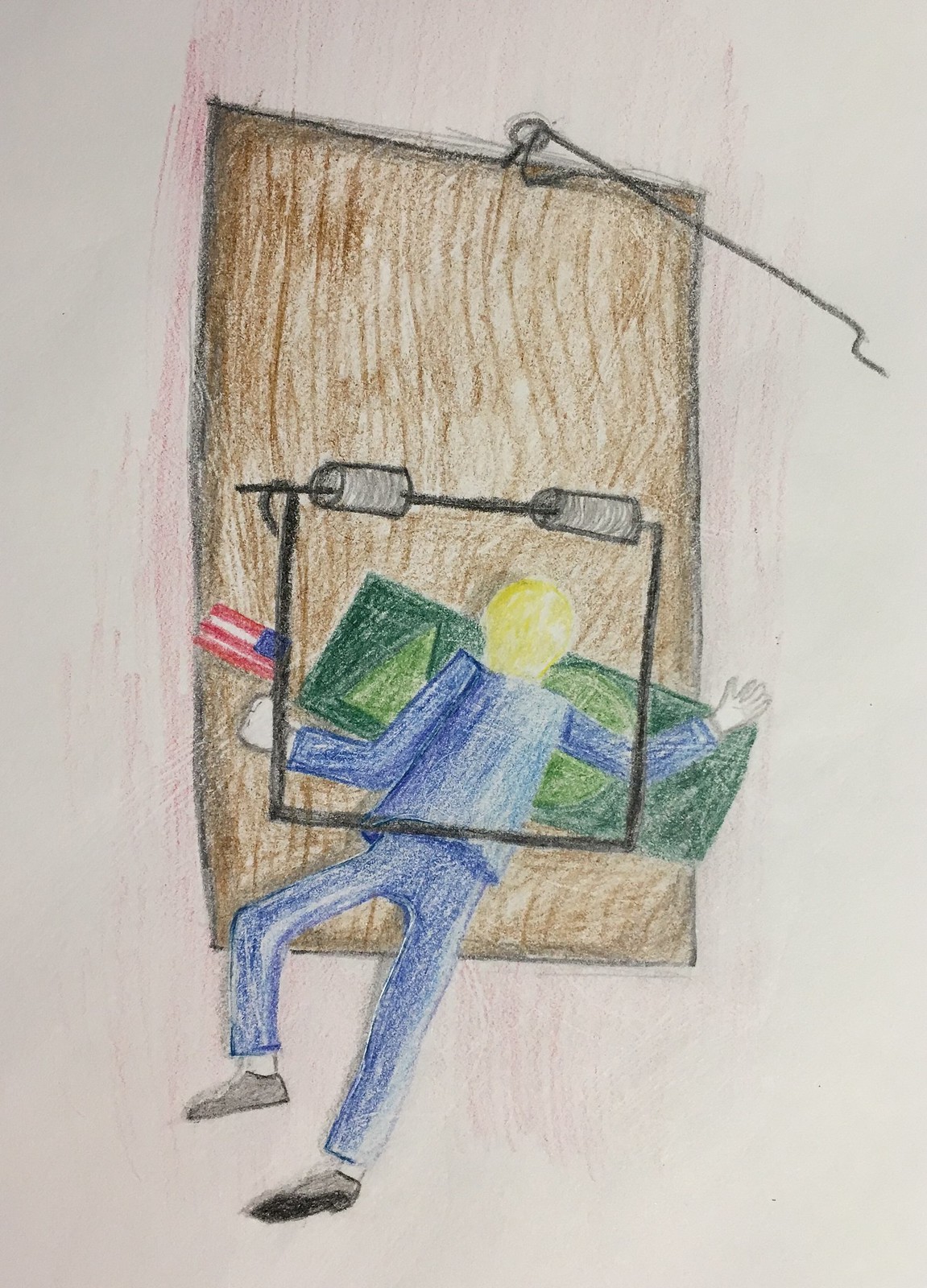Displayed in portrait orientation on a white piece of paper, this colored pencil drawing vividly captures a sprung mousetrap. The mousetrap, rendered in shades of brown, is detailed with the wire mechanism prominently positioned at the top. Sprung and active, the trap has caught a man, who is depicted face down in a blue suit. His feet, clad in tan shoes, reveal a sense of motion stopped. Strikingly, the man has yellow hair and lies upon what resembles a dollar bill, although it’s merely a solid green surface shaped to imply money. To the side, an American flag is sketched in pencil, hinting at the theme of the illustration. The detailed and comic-like style suggests a commentary on the perils and entrapments of money.